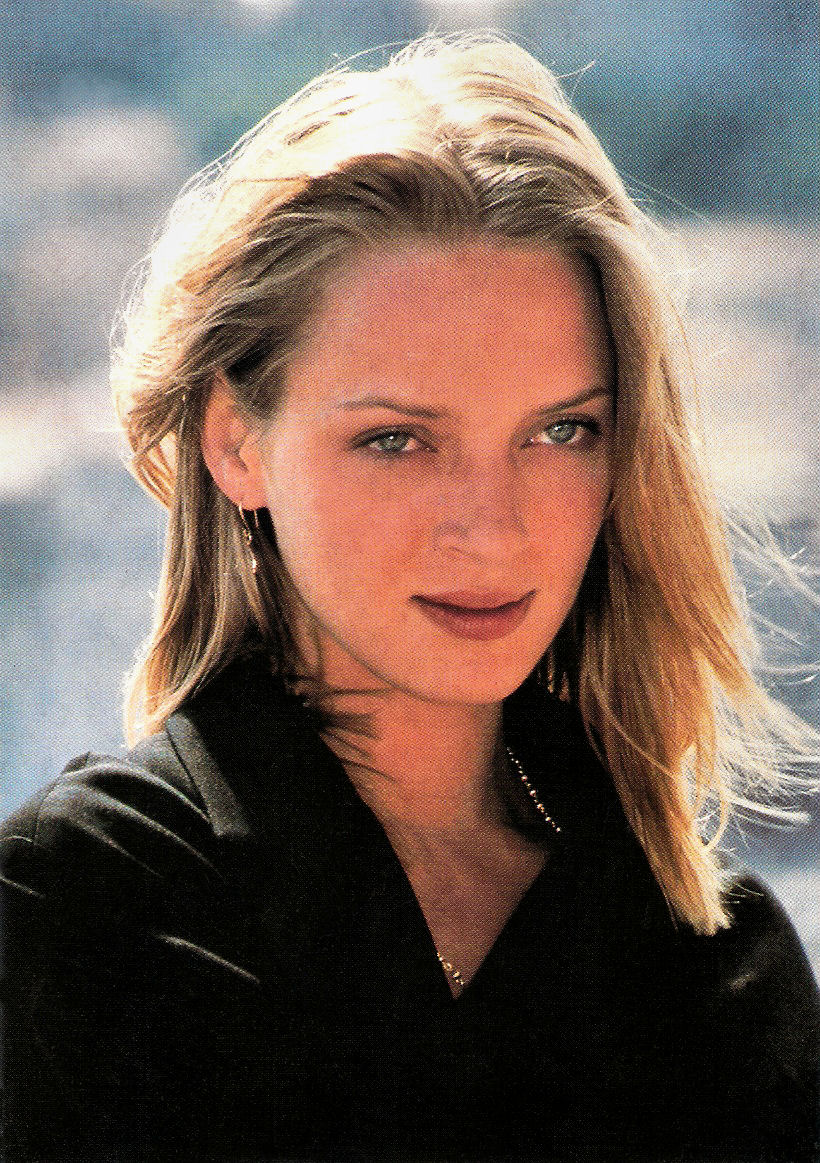This is a photo of Uma Thurman, likely taken during an outdoor shoot, characterized by its old, grainy, and low-quality appearance. Uma is wearing a black top and thin gold hoop earrings. She appears to be donning a gold necklace, partially obscured by her attire. Her hair is a light, golden-brown shade, shoulder-length, and gently windswept, adding a sense of movement to the image. Her expression is somewhat contemplative, with blue-green eyes gazing into the distance while her head is slightly tilted down. The background is a blurred mix of whites and blues, making it indistinguishable but emphasizing the outdoor setting suggested by her windswept hair.